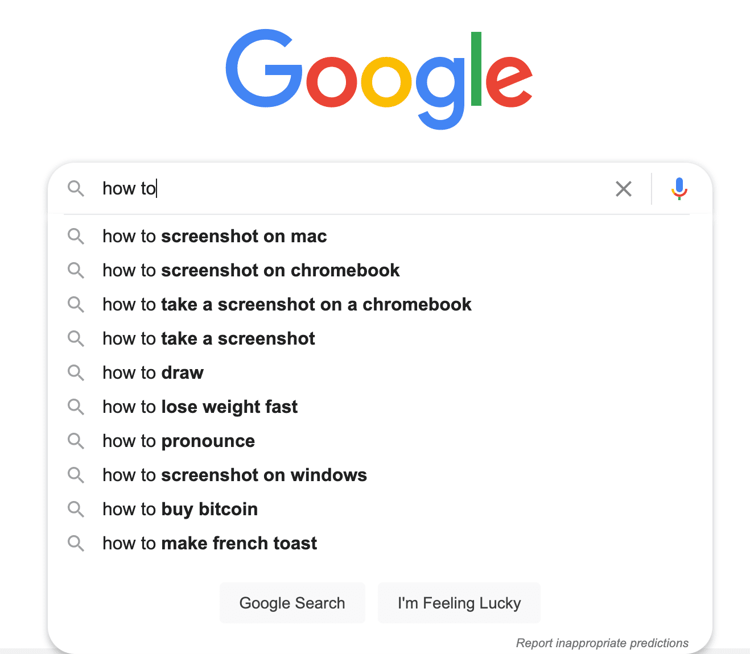The image displays a Google search page featuring the iconic Google logo at the top, with the letters colored in blue, red, yellow, blue, green, and red, respectively. Below the search bar, which contains the partially-typed query "how to," there is a list of autocomplete suggestions. These suggestions are arranged in a vertical, left-aligned format and include:

1. How to screenshot on Mac
2. How to screenshot on Chromebook
3. How to screenshot on a Chromebook
4. How to take a screenshot
5. How to draw
6. How to lose weight fast
7. How to pronounce
8. How to screenshot on Windows
9. How to buy Bitcoin
10. How to make French toast

Each suggestion is accompanied by a clickable magnifying glass icon to its left, allowing users to execute the search. 

At the bottom center of the page, there are two primary buttons: "Google Search" and "I'm Feeling Lucky." Just below these buttons, on the far bottom right, there is an option labeled "Report inappropriate predictions."

In the top right corner of the screen, there is a microphone icon colored in blue and red and an 'X' button.

The entire interface appears to be a clean and typical Google search page layout with no search results displayed, indicating that no search has yet been executed. The focused text input shows the beginning of a search query, suggesting a user is in the process of typing.